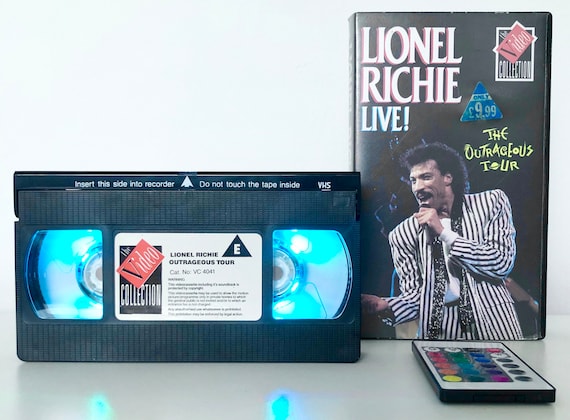In the photograph, three main objects are arranged on a glossy white table against a flat white wall. On the left, a VHS tape sits on its side, displaying lit-up blue rolls of tape behind clear plastic panels. The cassette is labeled "Lionel Richie Outrageous Tour" in black text across a white rectangle, also featuring a black triangle with a white "E" and another triangle with the words "The Video Collection," including a small red triangle behind the word "video." At the top, white text instructs, "Insert this side into recorder," accompanied by an upward-pointing arrow and the cautionary note, "Do not touch the tape inside."

To the right of the VHS tape is its corresponding box cover, predominantly black with a vibrant image of Lionel Richie in a black-and-white pinstripe suit, holding a microphone with his left hand. At the top, "Lionel Richie" is printed in white text, with "Live!" in pink and white with an exclamation point. The box also features a logo for "The Video Collection" in the upper right, near a blue triangle boasting "Only £9.99." Below, in striking yellow text, it says "The Outrageous Tour."

Positioned at the bottom right corner of the frame, a flat white rectangular remote control sits on the table, designed for RGB lighting strips. The remote is adorned with various colored buttons—white, red, orange, yellow, green, blue, dark blue, and purple—indicating color options for changing the lights, seemingly matching the blue LED lights embedded within the VHS tape.